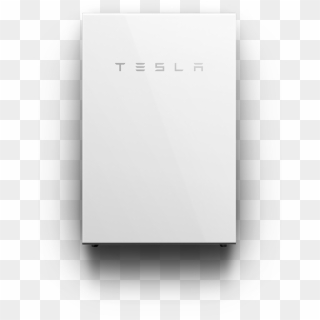The image is a screenshot that prominently features a white, cubic-shaped box rendered in a 3D perspective, complete with visible sides and shadows to accentuate its dimensionality. Emblazoned across the front of the box is the iconic Tesla logo, presented exactly as the company stylizes it: a capital "T," followed by an "E" comprised of three horizontal lines, an "S," an "L," and an "A," sequentially spelling out "TESLA." The backdrop consists of a gray and white checkerboard pattern, reminiscent of a background typically seen in image editing software when an image's background is transparent or being filtered out. The scene is minimalistic, with the checkerboard expanse and the prominently placed Tesla box being the sole visual elements, underscoring the box's centrality in the composition.